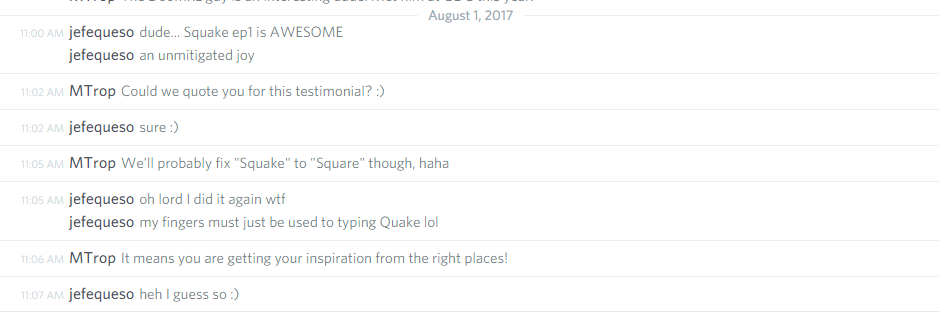This is a screenshot of a chat thread or forum post dated August 1st, 2017. The interface features a white background with dark gray text. The conversation is between two users: F. A. Queso and M. Tropp. Each message is timestamped, with the first entry beginning at 11:00 AM.

- **11:00 AM** - F. A. Queso: "Dude, Squeak episode 1 is awesome. It's been an unmitigated joy."
- **11:01 AM** - M. Tropp: "Could we quote you for this testimonial? :)"
- **11:02 AM** - F. A. Queso: "Sure."
- **11:03 AM** - M. Tropp: "We'll probably fix Squeak 2 Square though. And then, this is, oh lord I did it again, DmTF. My fingers must be just used to typing Squeak, LOL."

The chat highlights user interactions discussing the positive reception of "Squeak episode 1" and a humorous typing error by M. Tropp.